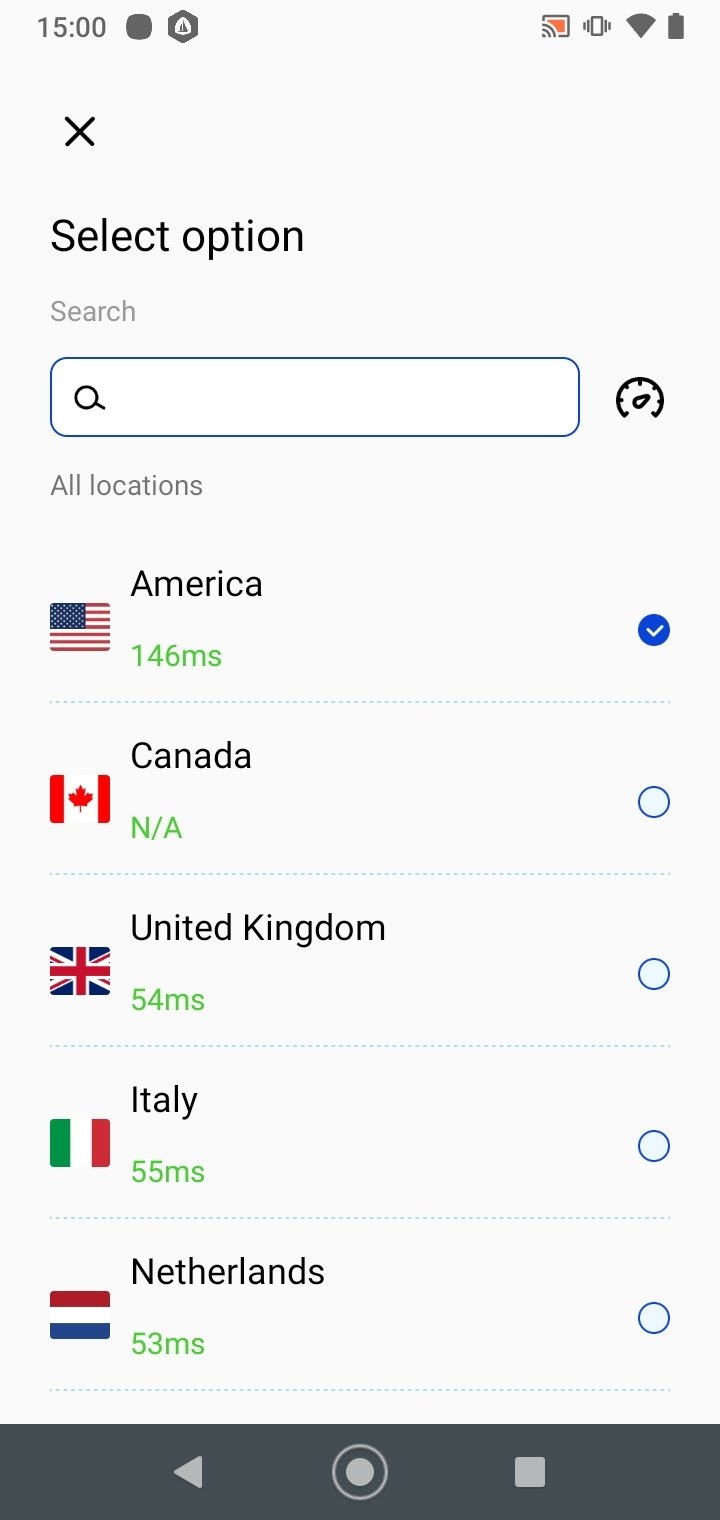Screenshot of a mobile app interface where users can select a location. At the top of the screen, there's an 'X' button for closing the menu. Below it, the text "Select Option" is followed by a "Search" prompt and a search bar iconified with a magnifying glass. Further down, the section titled "All Locations" lists various countries:

1. America (flag), 146 ms latency, with a blue checkmark indicating selection.
2. Canada (flag), N/A, with an available but unchecked circle.
3. United Kingdom (flag), 54 ms latency, with an available but unchecked circle.
4. Italy (flag), 55 ms latency, with an available but unchecked circle.
5. Netherlands (flag), 53 ms latency, with an available but unchecked circle.

At the bottom, there's a grey bar featuring a play button, a record button, and a stop button, indicating options for media control.